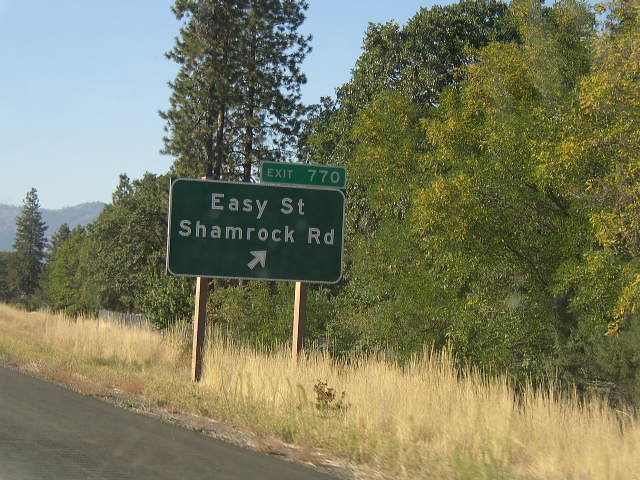A picturesque scene captures a serene landscape transitioning towards autumn. In the foreground, there is a strip of black asphalt forming a highway, bordered by dry, golden grass. The backdrop features a vibrant blue sky and majestic mountains towering in the far distance. A row of lush green trees, some with hints of yellowing leaves signaling the onset of fall, lines the landscape. Two particularly tall trees stand prominently together, adding to the natural beauty of the scene. By the side of the highway, a green sign with white lettering is supported by wooden legs. The top of the sign reads "Easy Street," followed by "Shamrock Road" with an arrow pointing to the right, and "Exit 770" prominently displayed at the top right corner. The scene is bordered with dry grass alongside the road, completing this seasonal transition image.